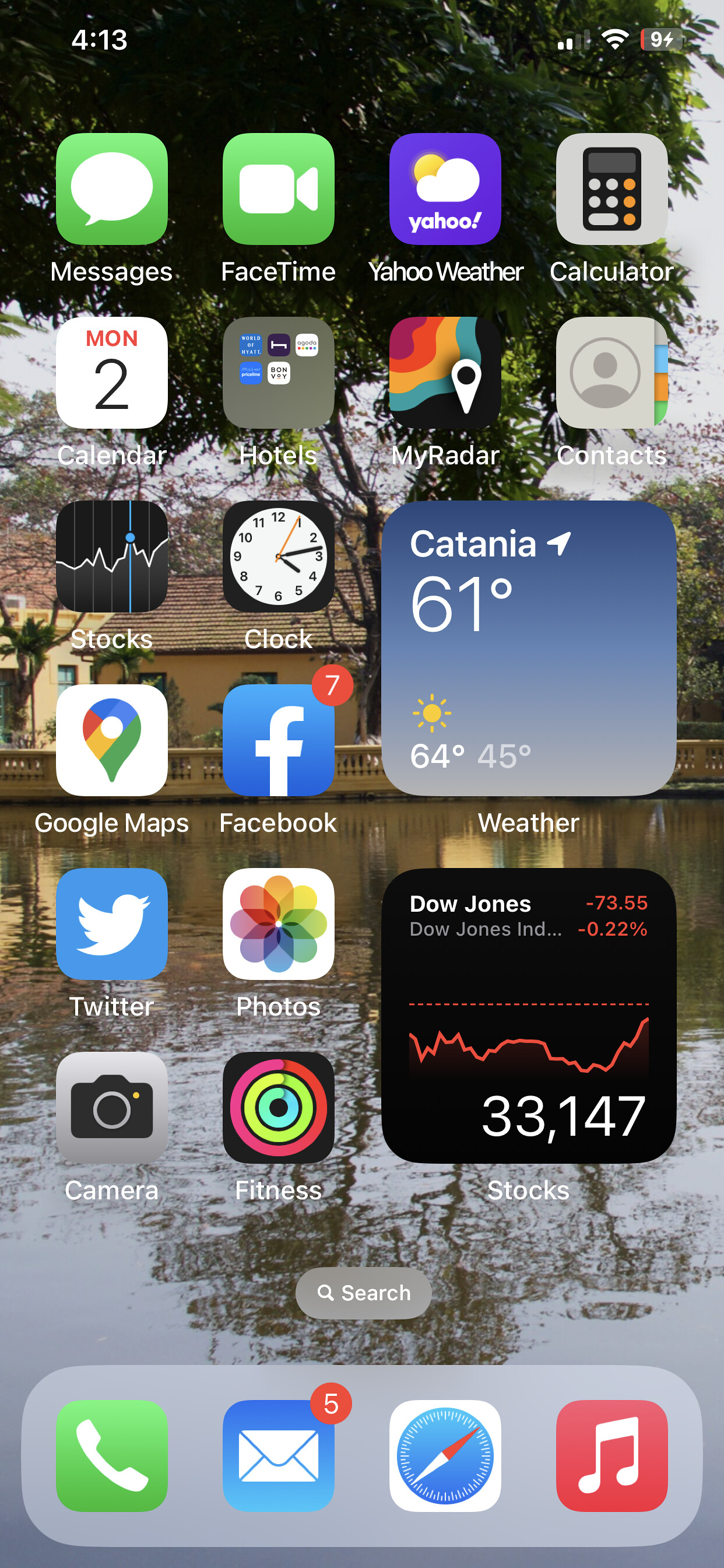This image captures the home screen of an iPhone, densely populated with a variety of apps from top to bottom. At the top status bar, the time is displayed as 4:13. The signal strength is indicated by two bars, and full WiFi connectivity is shown. The battery icon, featuring a lightning bolt, shows a charge level with the number 9 inside it.

The apps visible on this home screen include Messages, FaceTime, Yahoo Weather, Calculator, Calendar, Hotels.com, MyRadar, Contacts, Stocks, Clock, Google Maps, Facebook, Weather, Twitter, Photos, Camera, Fitness, and a second Stocks app. At the bottom of the screen, a search option is present, along with a dock holding four additional apps: Phone, Mail, Safari, and Music.

The background photo features a scenic view dominated by a large tree and a body of water. Between these elements is a building, partially obscured by a railing. The primary colors in the background are shades of green and blue, contributing to a serene and picturesque backdrop for the varied and colorful app icons.